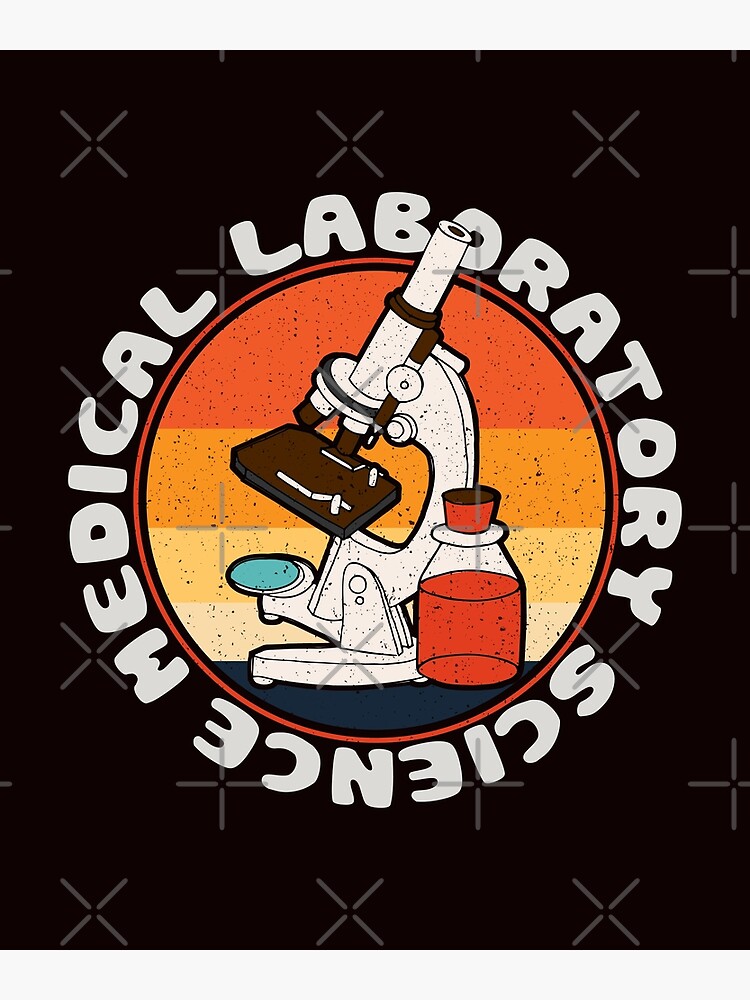The image is a retro-styled vector graphic featuring a central cartoon drawing of a microscope, without a slide or an aperture, but with a mirror at the bottom. Adjacent to the microscope, to its right, is a bottle filled two-thirds with red liquid and sealed with a red cork, slightly hovering above a dark blue or black table. The background transitions through a gradient from red at the top, to orange, yellow-orange, and pale yellow towards the bottom. Surrounding the central image, the text "Medical Laboratory Science" is arranged in a cyclical, bubble-letter format. The entire graphic has an overlay of repeating plus and X symbols, made of four unconnected lines, serving as a watermark. The overall aesthetic conveys a logo-like appearance, emphasizing a vintage vibe with a gradient-colored circular backdrop.